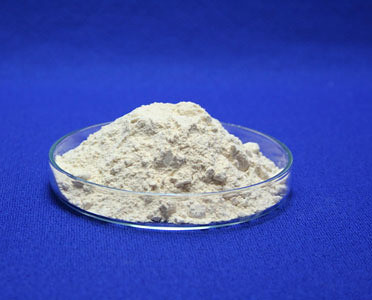The image depicts a clear glass petri dish set against a royal blue, textured background, which resembles cloth. The dish is filled with a noticeable amount of off-white powder, likely baking flour, though it could plausibly be dried plaster or another similar substance. The powder isn't finely milled, exhibiting visible clumps throughout, and it forms a small mound that rises above the rim of the dish. The setting is simple, focusing solely on the petri dish and its contents, presented within a nearly square frame.